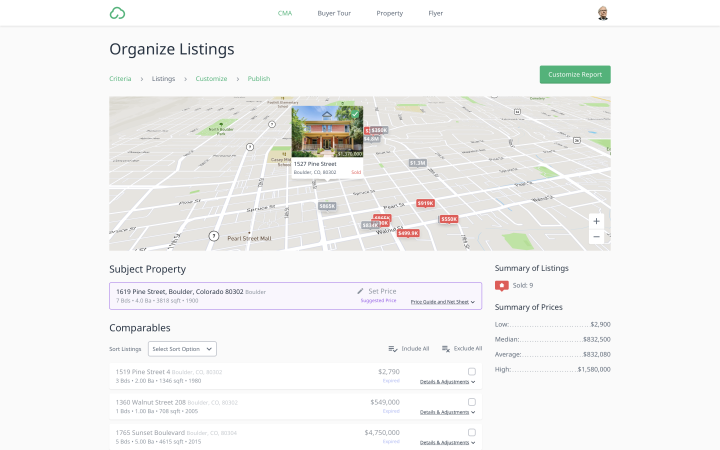The webpage displays a detailed property listing interface. The top row features a white background, with the upper left corner adorned by a white cloud icon outlined in green. To its right, four navigation options are present: "CMA" highlighted in green, followed by "Buyer Tour," "Property," and "Flyer." On the far right, a circular avatar of a smiling Caucasian male is visible.

Directly below, a light gray section reads "Organized Listings" in black text. This section includes a navigation path with arrows indicating "Criteria," "Listings," "Customized," and "Publish." The "Listings" option is highlighted in gray, while green highlights indicate the remaining options. On the far right, a significant green button displays "Customize Report."

The main interface features a detailed map showcasing a city layout, marked with white roads, gray buildings, and green park areas. Central to the map are gray squares with white numbers and orange squares with white numbers, highlighting property listings. A preview image of a selected property, a pink two-story home with columns, a front porch, surrounding green trees, and a blue sky, is visible. The preview's white bottom section includes the address "1527 Pine Street, Colorado," accompanied by an orange number, though finer details are difficult to decipher.

Below this map section is the "Subject Property" section. It displays a purple-highlighted box with the address "1619 Pine Street, Boulder, Colorado, 80302," and additional unreadable text. Below, there are various percentages with unreadable values and a "Set Price" feature. Additionally, there's a dropdown menu with indistinguishable text.

The "Comparables" section follows, allowing users to start listings and select sort options. Three properties are listed:

1. "1519 Pine Street" for $2,790,000, featuring three bedrooms, two bathrooms, 1,346 square feet, built in 1960-something. A checkbox and unreadable black text are adjacent.
2. "1360 Walnut Street, Unit 208" priced at $549,000, with one bedroom, one bathroom, and 700 square feet, built in 2005. Similar checkbox and text placement apply.
3. "1765 Sunset Boulevard, Boulder, Colorado" listed at $4,700,000, boasting five bedrooms, five bathrooms, 4,815 square feet, constructed in 2015. An associated checkbox and unreadable text are present.

The final section, "Summary of Listings," on the far right, features a red square indicating something related to "sold nine." Below is the "Summary of Prices" displaying a low of $2,900, a median of $832,500, an average of $832,080, and a high of $1,580,000.